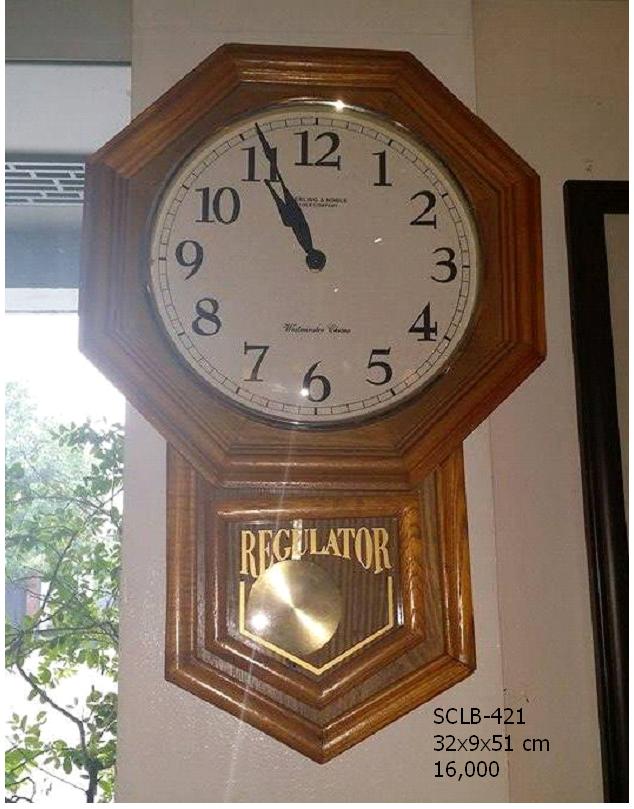This indoor photograph showcases a vintage wall clock, reminiscent of early 90s design, prominently displayed against a plain background. The clock is crafted from oak wood and has a unique octagon shape housing a round clock face with a beige background and bold black block numbers. The time displayed is 10:55 AM. The brand name "Westminster" is partly visible beneath the clock hands.

Adding to its intricate design, the lower section of the clock forms a triangular point, featuring a brass-colored pendulum disc that swings back and forth, enhancing its classic charm. A clear glass panel encases the pendulum, with the word "Regulator" elegantly inscribed on the glass.

In the lower right corner of the image, there's a text that reads "SCLB421 32x9x51 cm 16,000", likely indicating a model number, dimensions, or a price, providing an additional layer of detail to this nostalgic timepiece. The overall composition of the photograph highlights the fine craftsmanship and timeless appeal of the clock.